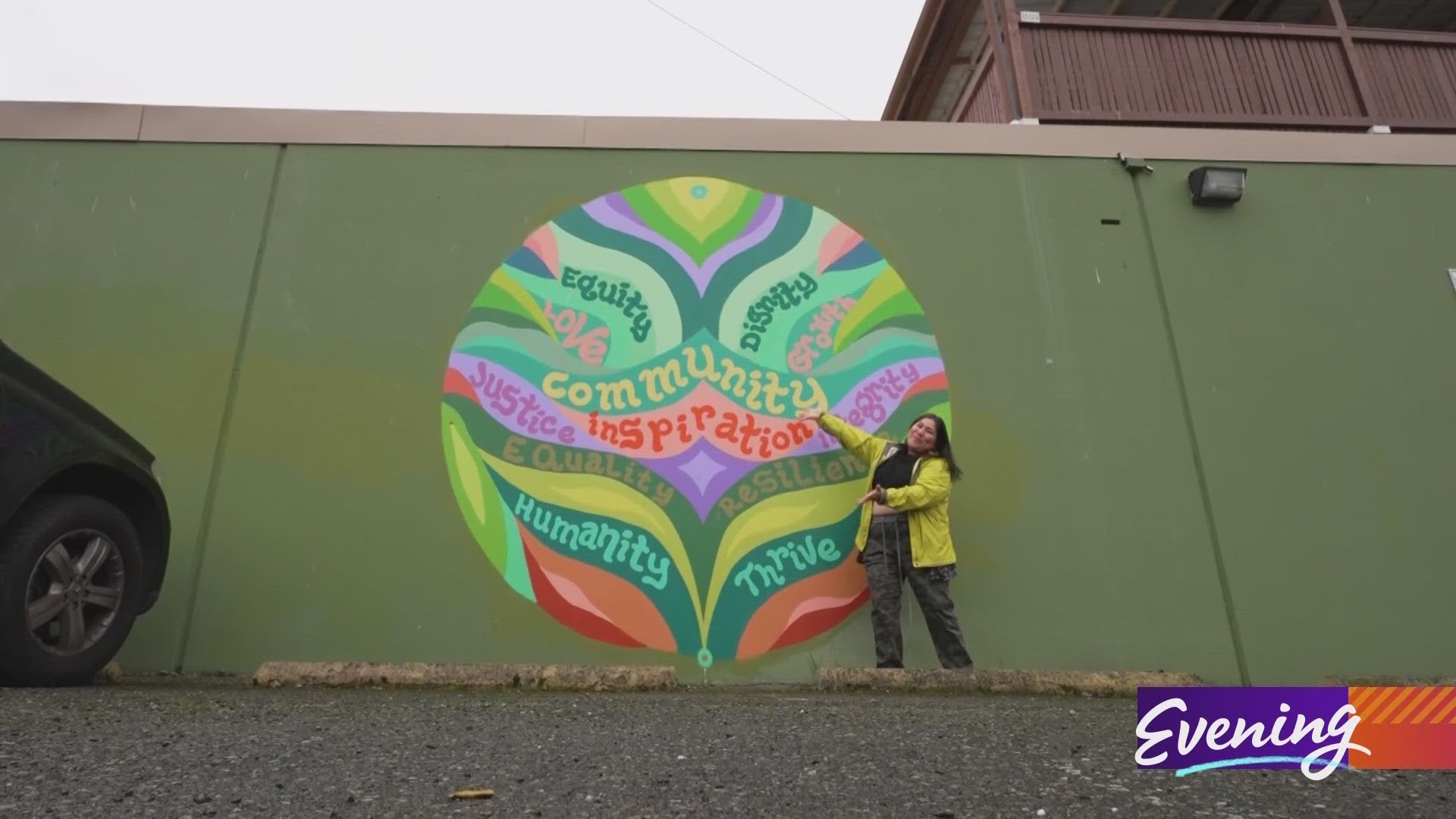This outdoor daytime photograph captures a detailed scene featuring a tall olive-green concrete wall with a brown border at the top. Dominating the center of the wall is a vibrant, round mural with symmetric rainbow-colored stripes in a psychedelic pattern. The mural displays inspirational words such as equity, dignity, love, growth, community, inspiration, justice, integrity, equality, resilience, humanity, and thrive. At the lower left and right, the image shows a gray pavement with small rocks and low concrete parking borders, with the front nose and tire of a black vehicle visible on the left side of the frame. A woman, possibly of Native American descent, with long black hair parted at the center, is standing to the right of the mural. She is wearing a yellow jacket, a black shirt, and camo pants, smiling with her arms outstretched towards the mural. In the lower right-hand corner, the word “Evening” in white cursive is overlaid on a purple and orange background. The top left of the image reveals a gray sky, while the top right shows the edge of a brown building.